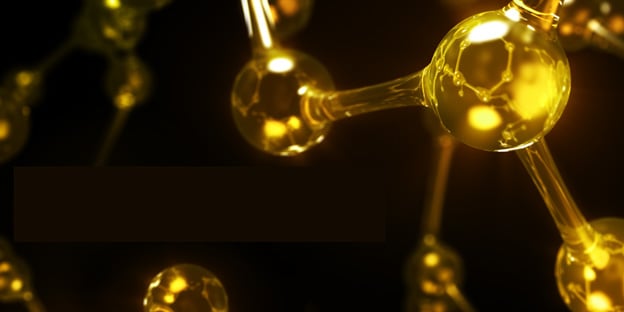This image is a very detailed, close-up photograph of molecular models set against a black background. The models consist of round, yellow, translucent spheres representing atoms, which are interconnected by thinner lines or rods of the same material. The primary focus is on a prominent, well-lit sphere in the foreground, which appears somewhat illuminated and intricate, while several similar spheres recede into the blurred, dimly lit background, creating a sense of depth. The spheres have a shiny, gelatinous appearance and seem to reflect one another, forming a network that appears fluid and dynamic. The entire arrangement resembles a 3D visual representation of molecules, emphasizing light and movement within the molecular structure.